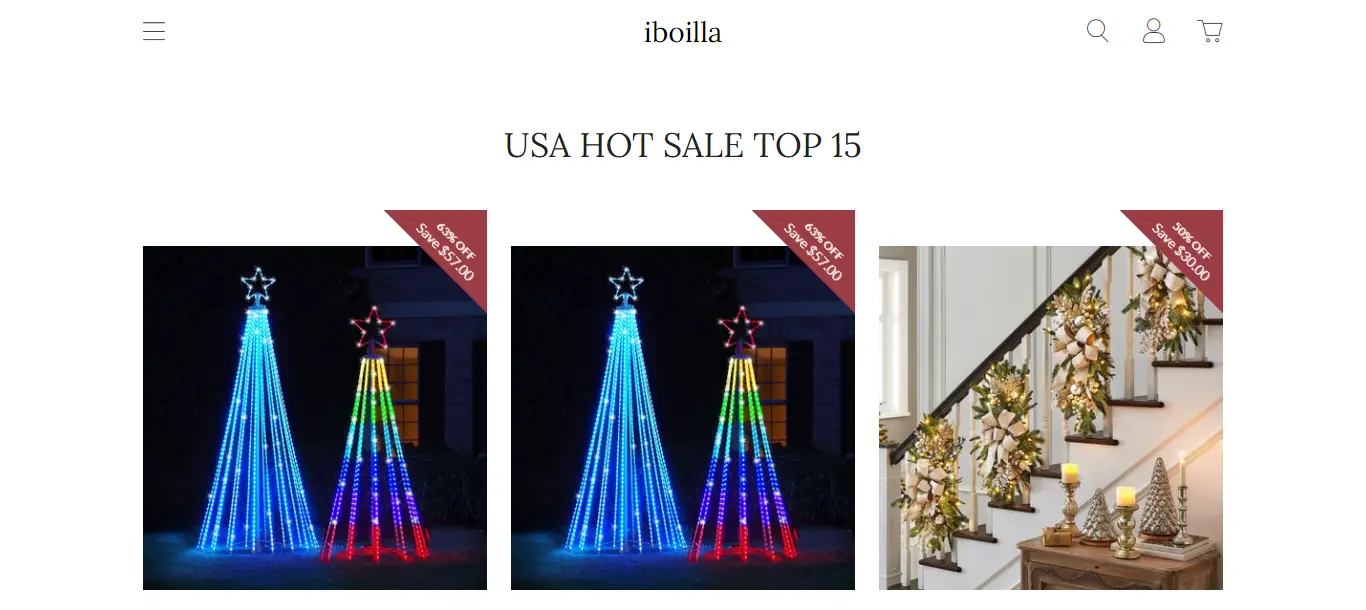This webpage showcases a festive holiday sale. At the top center of the page, the brand name "IVOILLA" is displayed in bold black letters. The left side of the header features three horizontal black lines, commonly indicating a menu or navigation option. On the right side, there are three icons: a magnifying glass for search functionality, a silhouette of a person likely signifying account login, and a shopping cart for purchases. Below the brand name, the text "USA Hot Sale Top 15" is prominently displayed in bold black font.

On the left-hand side of the page, there are two identical photographs. These images feature a decorative laser light tree, the first of which has cyan blue lights with a white star on top and dark blue lights at the bottom, casting a blue hue onto the ground. The second tree, similar in design but shorter, has a red star on top and multi-colored LED lights transitioning from yellow at the top to green, cyan blue, dark blue, purple, and red at the bottom. The different colors cascade onto the ground, with cyan and dark blue casting a blue hue and yellow, green, blue, purple, and red casting a red hue. The background reveals a white house with black shutters and silhouettes of trees, illuminated by light streaming through the windows. A banner in the top right corner of these images reads "Save $57" with "63% off" above it.

On the right-hand side of the page is a festive banister adorned with white floral patterns, dark green leaves, and gold accents. The banister is decorated with candles and lights against a white wall, with an off-white wall in front of the door. There is a "50% off" banner in the top right corner of this section, indicating a $30 savings. Additionally, a small nightstand beneath the banister displays candles and miniature Christmas trees, enhancing the holiday cheer of the scene.